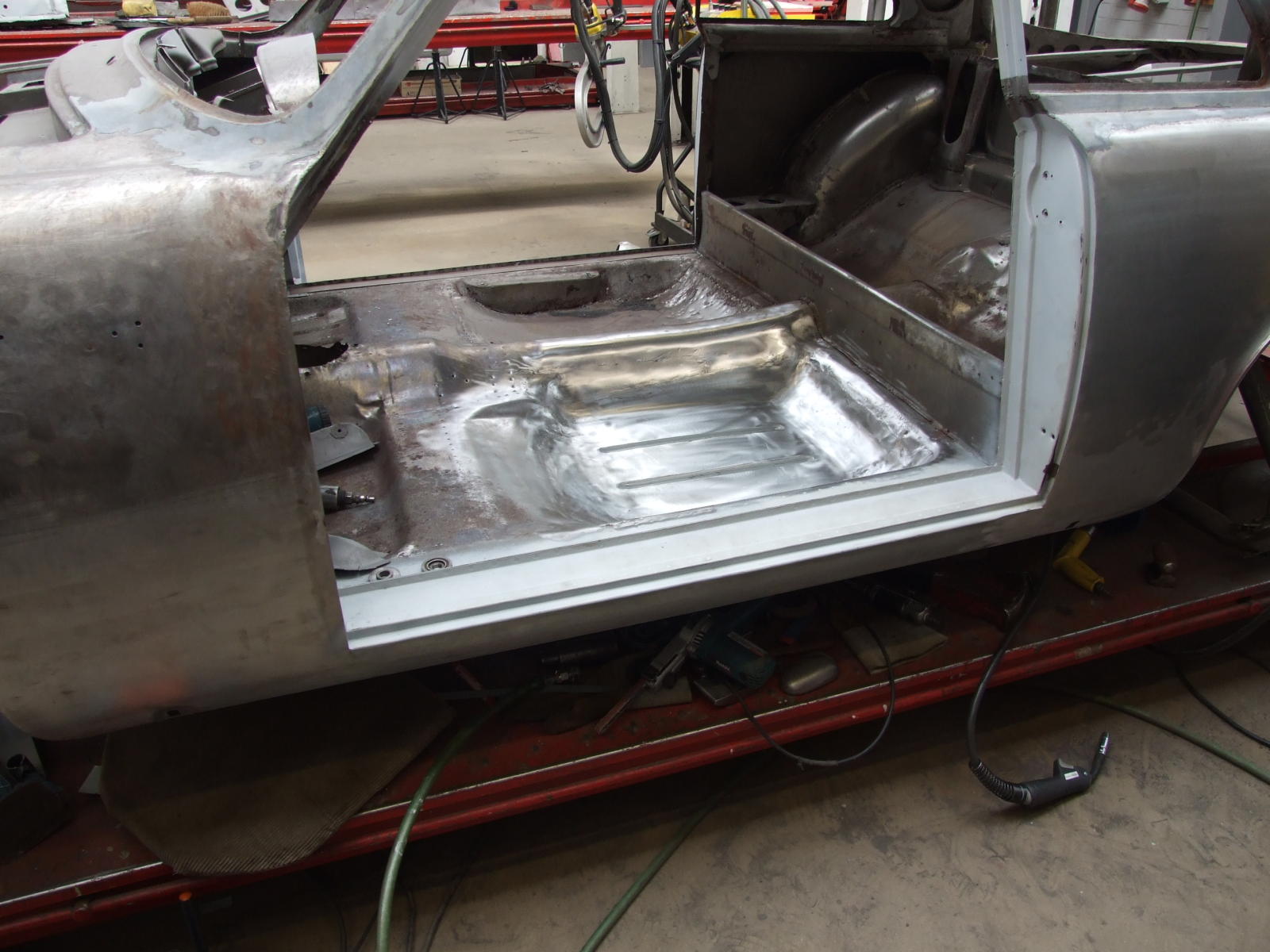The image showcases the stripped interior of an old, metallic silver vehicle undergoing extensive repairs inside a basic, no-frills body shop. The car, elevated on a red platform strewn with various tools, wires, and hoses, shows clear signs of soldering, grinding, and bodywork repairs around the windshield, floorboard, and console area. With the doors removed, fenders exposed, and the console area torn out, the car appears to be a work-in-progress, possibly being rebuilt or used for parts. In the driver’s and passenger’s footrest area, numerous tools are scattered, including an arc welding torch lying on the floor in front of the vehicle. Jack stands and more equipment can be seen lined up in the distance, reinforcing the ongoing nature of the work. The surrounding shop area is basic and functional, emphasizing utility over aesthetics, with cords and numerous tools hanging and scattered throughout, contributing to the industrial, work-in-progress atmosphere of the scene.